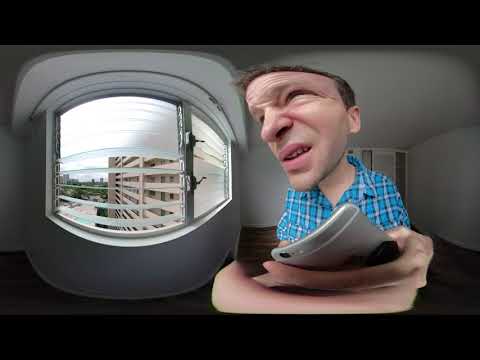The image depicts a humorous, distorted wide-angle photograph of a man with brown hair and a prominent nose, sitting in an unfurnished room with light gray walls and a brown wooden floor. The man, wearing a collared, plaid shirt in shades of blue, dark blue, and white, with rolled-up sleeves, is holding a gray iPhone. His facial expression is a mix between a smirk and a sneer, exaggerated by the lens distortion that enlarges his head and stretches his hands. To the left of the man is a large, semi-circular window with open blinds through which a tan apartment building and some green trees are visible. There is also a white ceiling, and a door can be seen over his left shoulder. The overall effect of the image is comical due to the warped perspective, making the man and parts of the room appear unusually shaped.